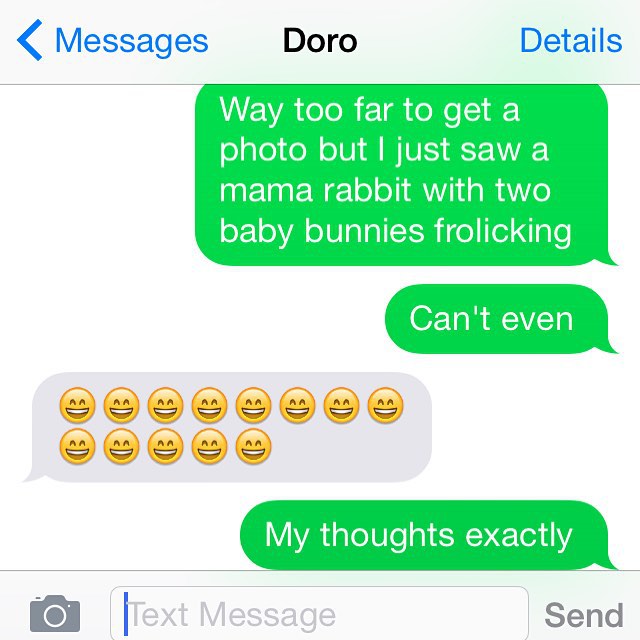This image is a screenshot of text messages on a phone between two people, displayed on a green background. At the very top of the screenshot, in blue text on a white background, is the word "Messages" with a back arrow pointing left. Centrally positioned is the name "Doro" (D-O-R-O) in black lettering, and on the upper right corner, a blue link labeled "Details".

The main body of the screenshot features the conversation. The first message is in a green chat bubble with white text that reads, "Way too far to get a photo, but I just saw a mama rabbit with two baby bunnies frolicking." Below it is a smaller green chat bubble with the text, "Can't even." The response from the other person is in a gray chat bubble containing twelve smiling face emojis, arranged in two lines. Following this, another green chat bubble reads, "My thoughts exactly."

At the bottom of the screenshot, there is a field for entering a new text message, accompanied by a camera icon on the left and a "Send" button on the right.